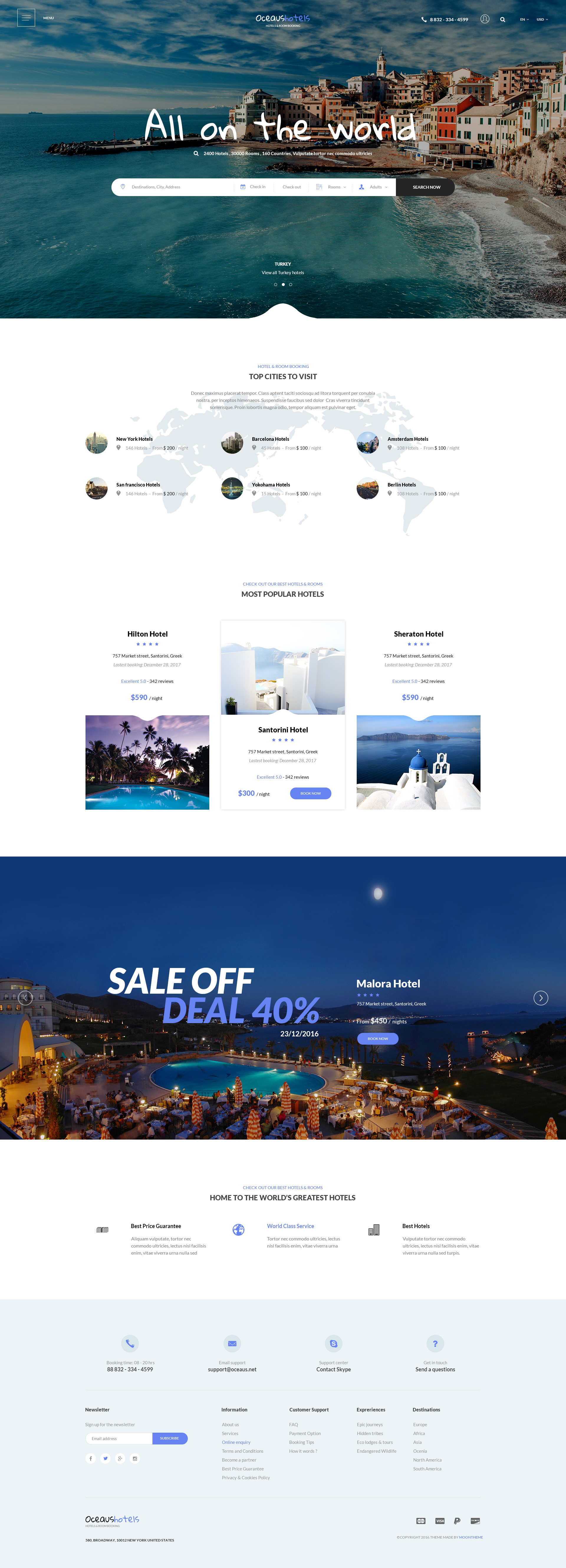This image displays a vibrant travel website named "All on the World." At the top of the page, the website’s title is prominently shown. The central section features a picturesque ocean scene with numerous apartments or hotels aligned along the shoreline, set against a backdrop of a blue sky speckled with clouds.

The navigation area is cluttered with various menu options, though the text is minuscule and illegible even when magnified. Below this, there is a box containing six choices, each accompanied by an oval picture and blue text describing the option, though the text remains too small to read clearly.

Further down, the webpage features four larger rectangular selections. The first image showcases vividly blue water with trees, including palm trees, and a deep blue sky. The middle section consists of a collage of several smaller images: one of clouds and trees, another of clouds alone, and a third depicting a shoreline view. The rightmost image presents boats in the water with a backdrop of blue water, a line of trees, and distant hills or mountains.

Dominating the page is a large banner stretching across the entire screen, loudly announcing "SALE, SALE OFF, 40% DEAL." This section features an evocative dusk scene with a yellow hotel building on the far left, a large blue oval-shaped swimming pool in the center, several other buildings, and trees. In the distance, water and possibly some islands are visible. The sky appears dark and cloudy with a bright white light that could either be a moonrise or a sunset, adding to the atmospheric quality of the image.

Beneath this, a white section contains three more unreadable selection options, followed by a prominent blue box with additional options, again marked by minuscule, unreadable text. Overall, the webpage appears dynamic and engaging, though hindered by the impractically small font used in many sections.